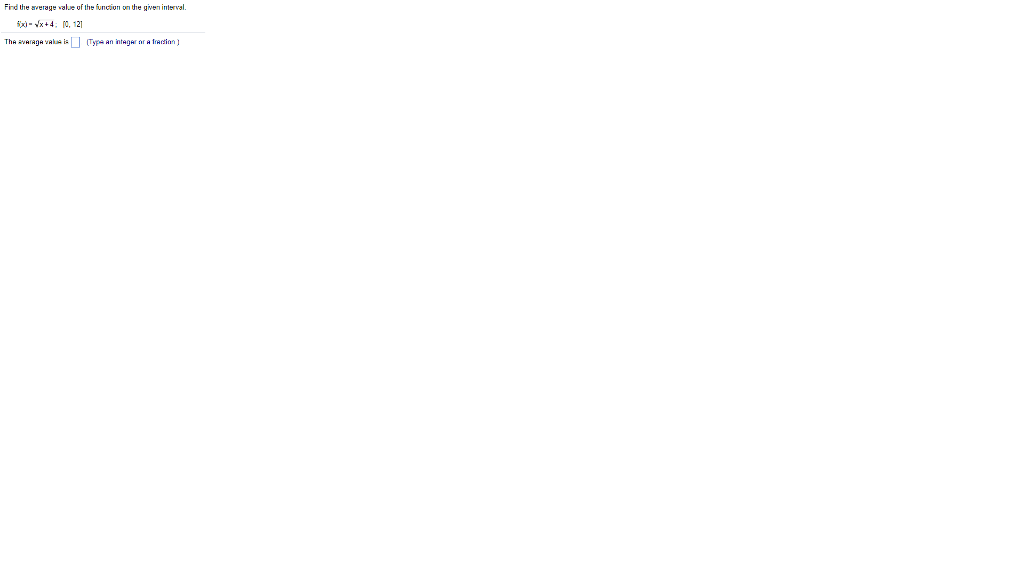The image predominantly features a large blank area. In the very top-left corner, there is minuscule black text accompanied by a thin horizontal line. Toward the bottom, a small box is visible. Upon enlarging the section, the text revealed appears to be a mathematical question from what could be a student's test. The instruction states, "Find the average value of the function in the given interval." Below this directive is an equation denoted as \( f(x) = \sqrt{x + 4} \). An additional text line beneath the equation reads, "The average value is," followed by a blank square where an answer is expected to be entered. The requirement is to type an integer or fraction in the provided box. The rest of the image remains unoccupied and devoid of any other significant details.